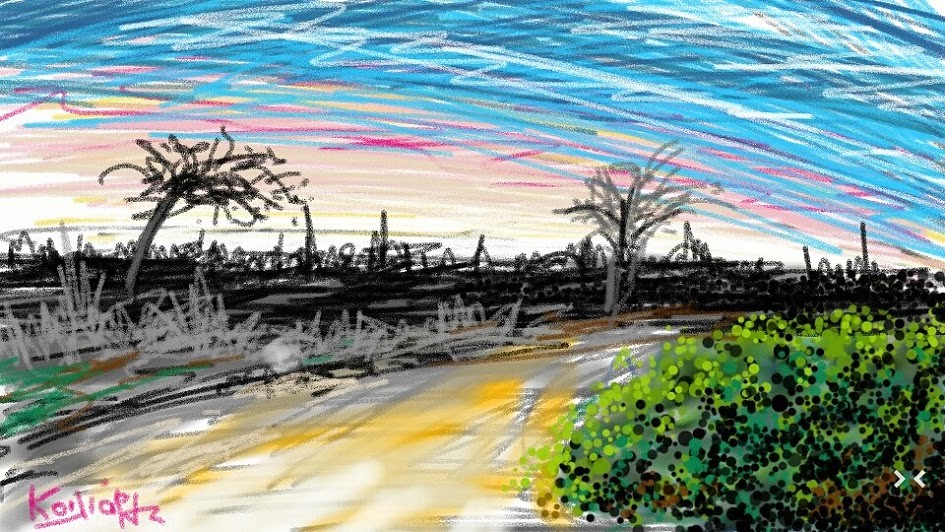This vibrant drawing portrays a forest scene with a notable contrast in appearance on either side of a narrow, dirt road. On the left side, the forest seems charred, with burnt trees rendered in black scribbles and pen dots, creating a sense of desolation. The road itself is marked with yellow and white paint strokes, adding texture and color variation. On the right side, the atmosphere brightens with a vivid green bush dotted with an array of colored circles, including shades of green, black, brown, teal, and light green. The sky above the scene is an eclectic mix of blues, pinks, and whites, illustrated in a dynamic, scribbled style. The artist’s signature, a scribbled name that appears to read "caulipots" or similar, is located in the bottom left corner, adding a personal touch to this imaginative and somewhat childlike piece of artwork.